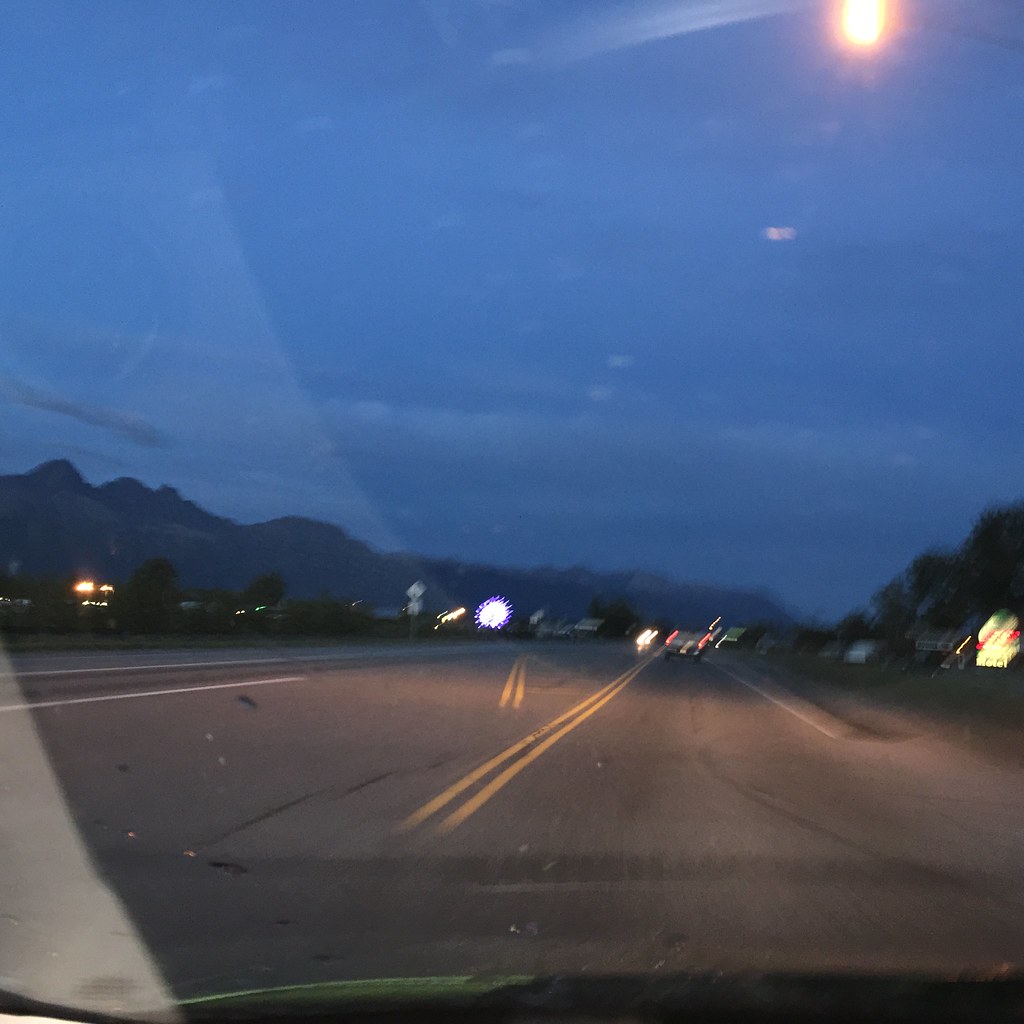This nighttime photograph captures a third-person perspective from within a moving car, driving along a highway around 8 pm. The scene is slightly blurry due to the motion, showcasing the car's windshield and part of the dashboard. The paved, black road in front is marked with yellow lines. Ahead, the blurry red brake lights of a truck are visible, along with the headlights of oncoming cars. To the left, dark blue mountains are silhouetted against a similarly dark blue sky. The horizon reveals some distant lit buildings and trees. Notably, there is a bright, white circular object with purple lines radiating from it, possibly a Ferris wheel or a casino sign, adding a sense of intrigue to the horizon.